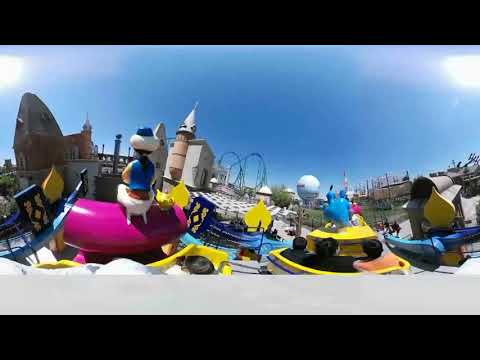The panoramic image captures a vibrant amusement park scene on a sunny day with a clear, blue sky. In the distance, at the center, are two loops of a roller coaster with elaborate tracks, adding excitement to the scene. To the left of the roller coaster, there's an ornate building resembling a castle with a turret, adding a whimsical element to the background. The park features various multicolored rides, including prominent yellow and blue carts, as well as a distinctive pink cart at the front with the back of an animated character sitting in it. The rides are interconnected and appear to move people around, with some carts brightly adorned with yellow and blue colors. There is a noticeable 360-degree warping effect in the photo, giving it a slightly distorted but playful appearance. The foreground showcases a row of carts filled with people enjoying the rides. Off to the left, there's a large figure resembling a genie, contributing to the park's animated and playful atmosphere. Verdant grassy areas surround the rides, enhancing the lively and colorful environment. In the far background, a structure resembling a giant golf ball can be spotted, hinting that the park might be a famous theme park like Disney World in Florida. Overall, the image conveys a joyful and immersive amusement park experience.